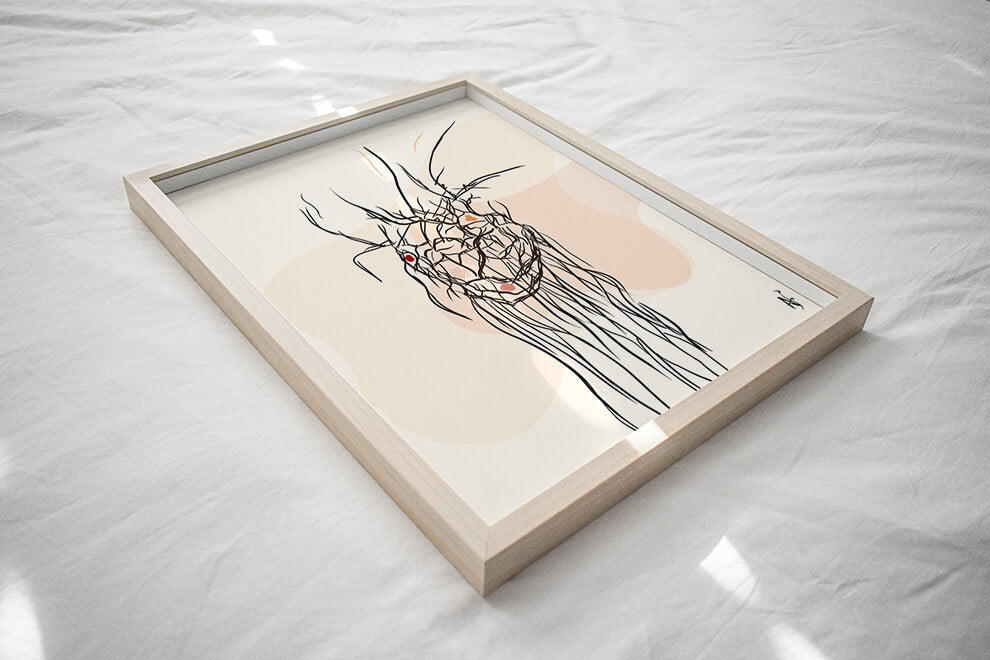A photograph captures a piece of framed, hand-drawn artwork resting on a bed covered with a white sheet, spreading across the entire background. The frame itself has a cream or sandy-colored border, transitioning to a white inner edge. The artwork inside showcases an abstract design comprised of numerous black lines running erratically, predominantly from top to bottom, complemented by red and pink spots. Upon closer inspection, the lines and colors create an undefined, possibly figurative or facial composition, set against a subtly shaded background that ranges from pale yellow to a slightly darker orange towards the center. The overall scene is softly illuminated by natural light, suggesting it is filtered through nearby curtains, enhancing the serene ambiance of the predominantly white environment.